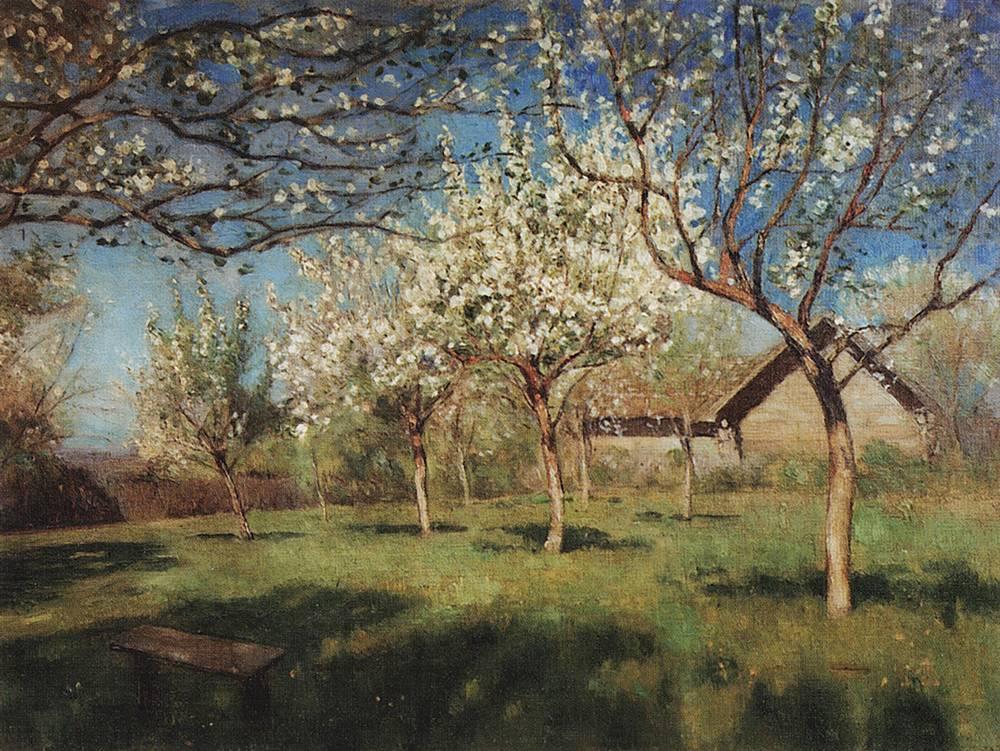The painting depicts a serene countryside scene with a small homestead in the background, featuring a peaked-roof structure to the left, seemingly made of wood with shingled roofing. In the foreground, a wooden bench is positioned in the shade, inviting viewers to sit and take in the tranquil surroundings. Multiple trees adorned with white blossoms—perhaps dogwoods—stand prominently, casting their shadows over a lush green field that stretches towards the distance. The sky overhead is a clear, vibrant blue, framing the entire composition. Brown grasses and earthy shades suggest a dirt path or plain extending out behind the trees and homestead, adding depth to the setting. The overall palette includes natural brown tones of the house and tree bark, contrasting with the bright green of the grass and the crisp white of the flowering trees, all rendered in a realistic oil pastel style, capturing a peaceful, sunlit daytime scene.